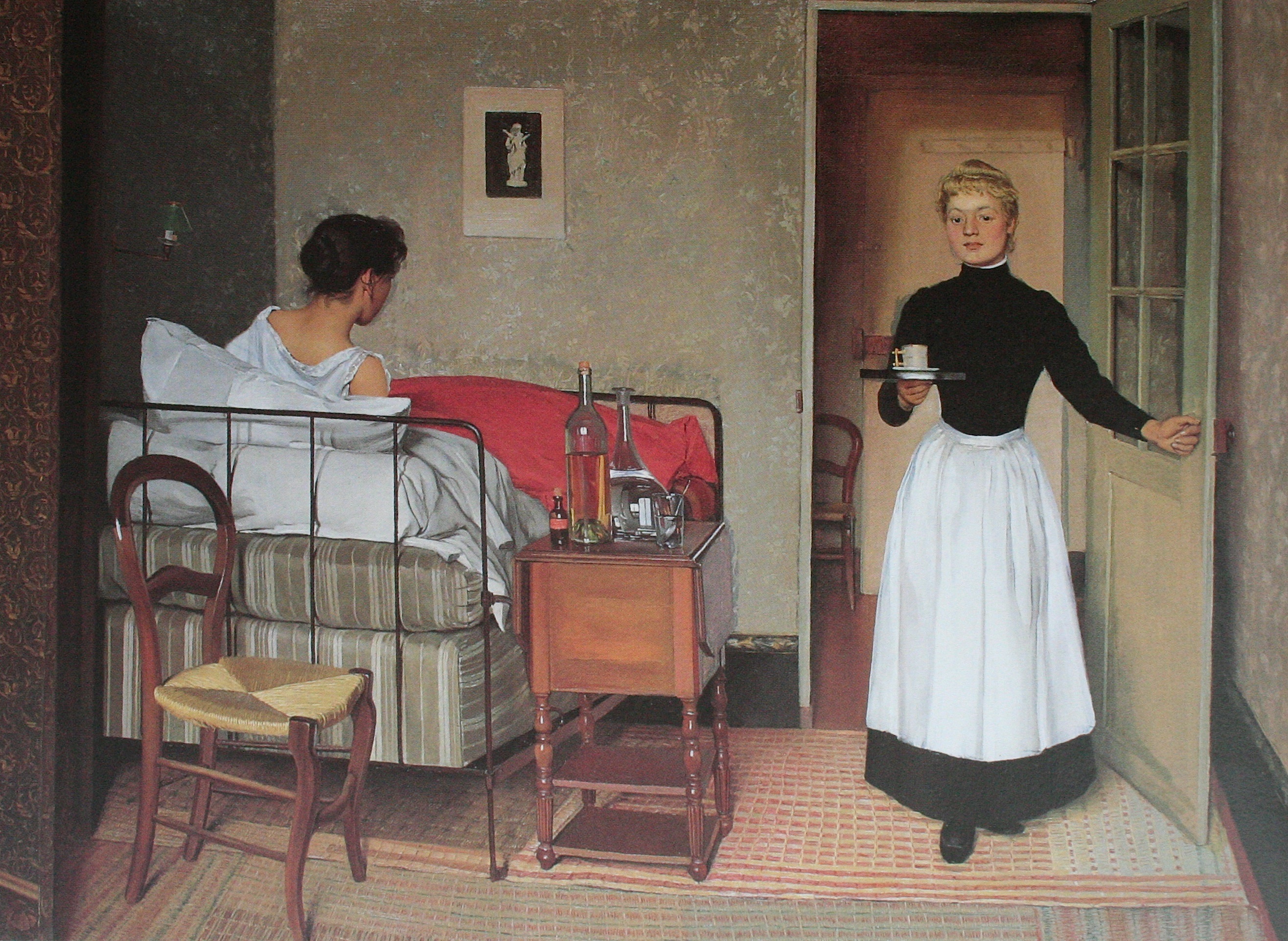In this color oil painting titled "The Patient" by Felix Vallotton, completed around 1900, a serene indoor scene unfolds. The focal point is a hospital room where a woman, likely a patient, reclines in a wrought iron daybed adorned with gray and white striped bedding and white pillows. She is dressed in a white nightgown and covered with a red blanket, her back turned towards the viewer as she gazes at the entering maid. The maid, positioned on the right side of the painting, is depicted in a traditional black dress with a white apron and collar, her blond hair neatly pulled back. She holds a tray with a white mug featuring a gold handle in her right hand, while her left hand remains on the doorknob, indicating she has just stepped into the room. To the patient's right, a brown table on wheels is cluttered with various bottles, some large and possibly containing water or wine, and others small, likely filled with medicinal liquids. Behind the patient stands a wooden chair with a woven straw seat, suggesting a place for visitors. The room’s backdrop includes grayish wallpaper adorned with a painting of a white statue. The floor has a pink or red rug, adding a touch of warmth to the otherwise subdued setting. The painting’s style blends avant-garde elements with realism, capturing a moment of quiet interaction and care.